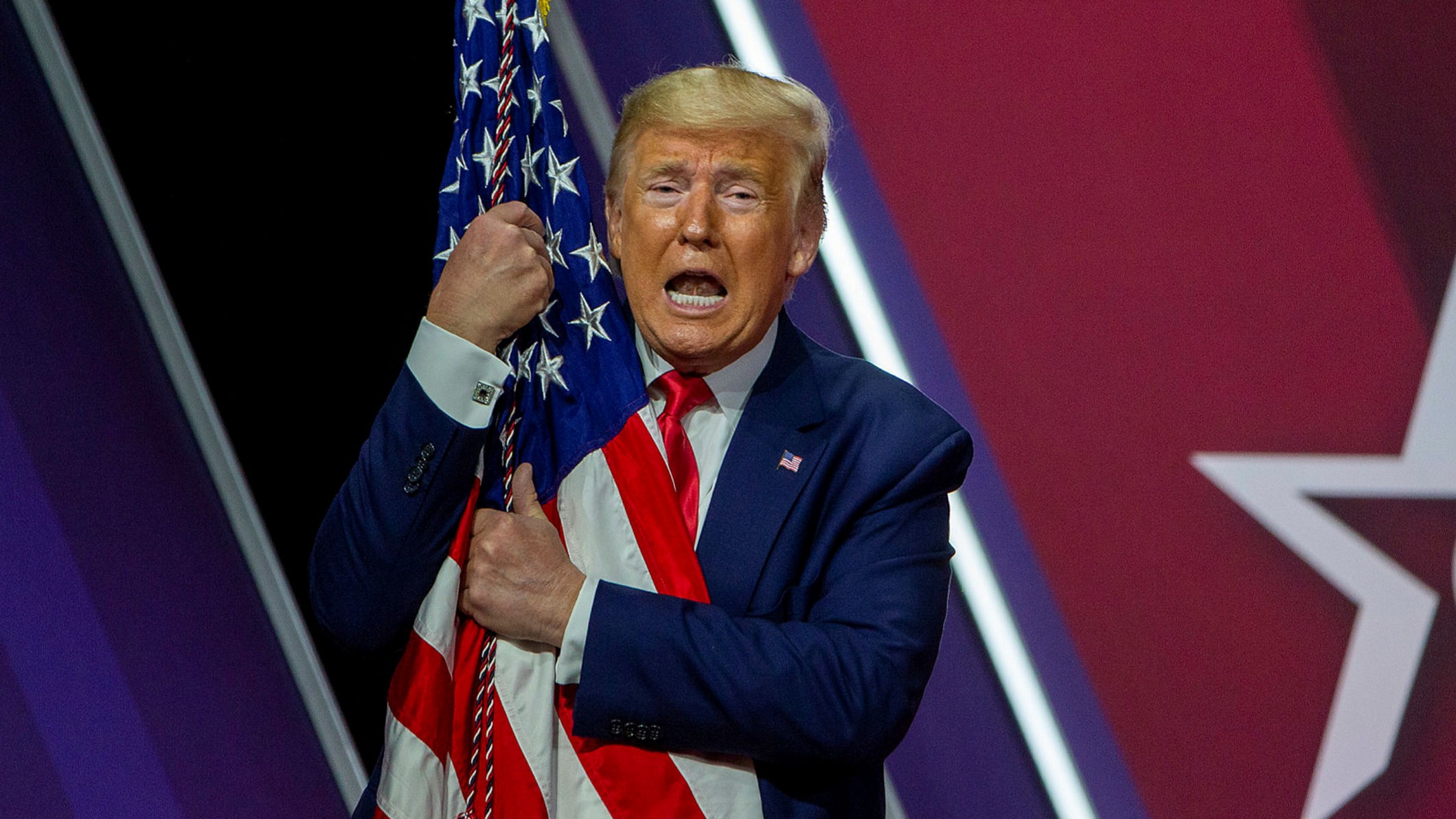In the image, former President Donald Trump, who is also running for president in the 2024 election, is seen clinging to an American flag mounted on a slim pole. The flag, proudly displaying its iconic red, white, and blue colors, stands out against a similarly colored background, creating a strong visual connection to American patriotism. Trump is dressed in a blue long-sleeve suit, accented with a button of the American flag on the lapel, paired with a red tie and a crisp white shirt. His mouth is open as if he is in the middle of speaking, though the exact words are unknown. With his left arm bent across his body, both of his hands firmly grasp the pole of the flag, displaying a gesture of fervent patriotism. His skin has a light tan with an orange tinge, while the area around his eyes and mouth is notably lighter, almost pale in comparison. His hair, a light blonde, lays somewhat flat with a characteristic swoop from left to right. The photograph is a striking portrayal of Trump, standing as the sole figure in the frame, firmly holding onto the symbol of the nation.